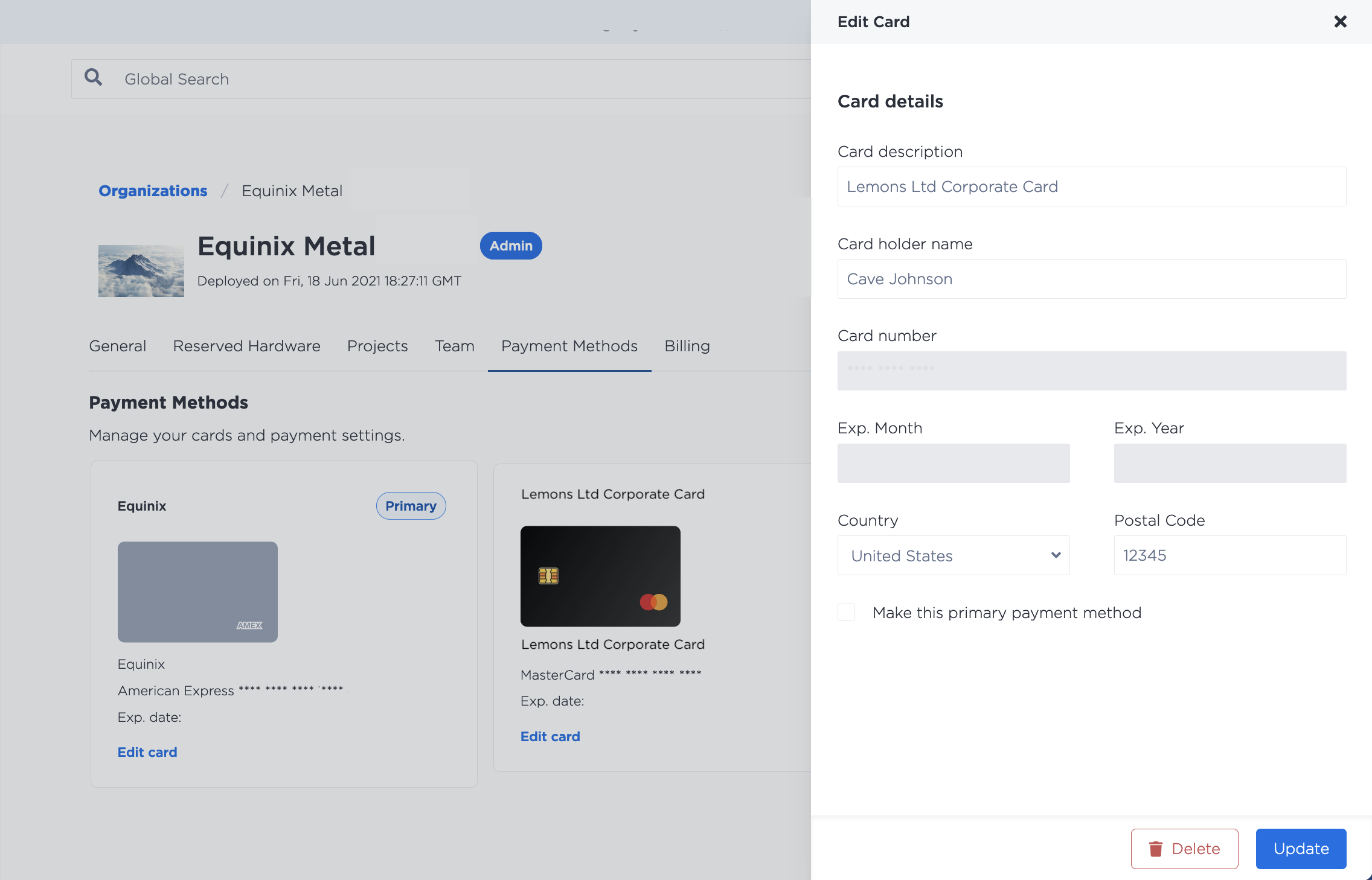**Description of the Screenshot:**

The screenshot is divided into two main sections. On the left side, there is a large gray square, while the right side features a more rectangular area with a white background. 

At the top of the left section, there is an indented search bar that contains a magnifying glass icon followed by small black text that reads "Global Search". About four lines down, there is a horizontal menu bar with the word "Organizations" in blue text, and next to it, "Equinix Metal" in black text.

Below this menu bar, on the left side, there is a square image of clouds. To the right of the image, the text "Equinix Metal" is written in bold black letters. Below this, some light gray text provides additional details, next to which there is a blue oval button labeled "Admin".

Continuing downwards, there is another menu with the following options: General, Reserved, Hardware, Projects, Team, Payment Methods (underlined in blue), and Billing. Below this menu, the section header "Payment Methods" is displayed in bold black text with a subtitle in gray: "Manage your cards and payment settings".

Two boxes are presented below this subtitle:
- The left box displays the text "Equinix" with a blue primary button to its right. Below this is an image of a card.
- The right box is titled "Lemons LTD Corporate Card" with an image of a credit card beneath it. At the top right of this box, there is an "Edit Card" option with an "X" beside it. The main content of this box includes the label "Card Details" in bold black. Form fields for card information are listed below: Card Description, Cardholder Name, Card Number, Expiration Month, Expiration Year, Country, and Postal Code.